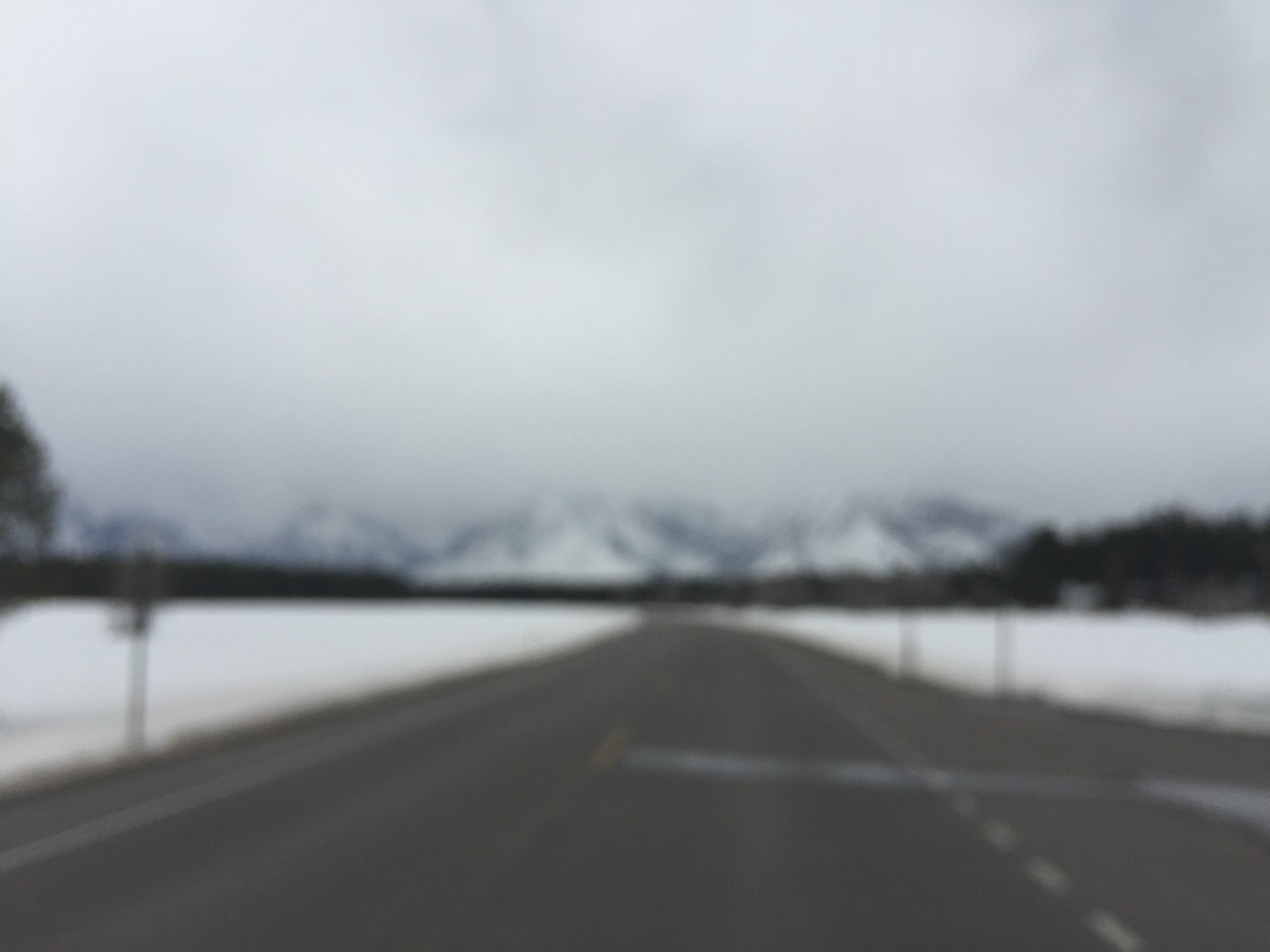This image captures a view of a winding highway leading towards majestic, snow-covered mountains that stand proudly at the horizon. The prominent white peaks of the mountains contrast starkly against a bleak, overcast sky, which casts minimal light over the landscape. On either side of the wet, glistening road, patches of snow blanket the ground, interrupted occasionally by rows of leafless trees. Sporadic posts and signposts line the roadside, hinting at civilization, but no houses are visible, giving the scene a remote and serene atmosphere. The overall mood is one of quiet solitude, heightened by the soft reflections on the damp pavement.